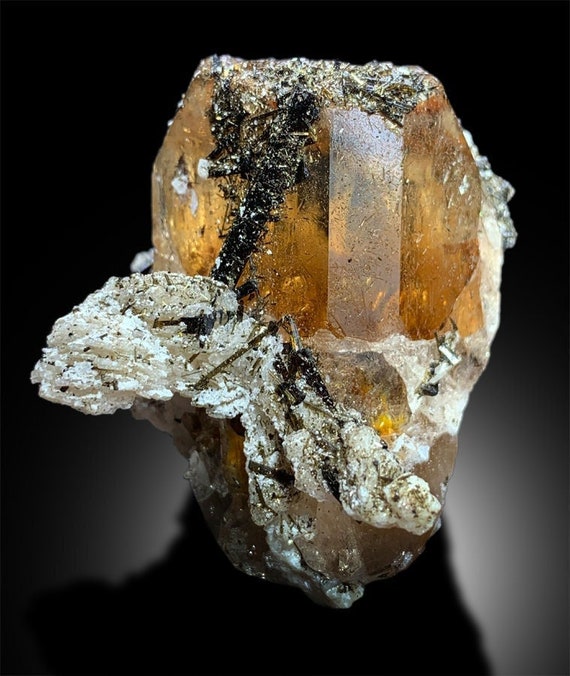This detailed color photograph in portrait orientation showcases an amber-brown topaz crystal situated on a black reflective surface, with a matching black background enhancing its appearance. The top portion of the topaz crystal is rounded and features faceted sides, exhibiting a shiny, clear, and well-lit visual quality. Some remaining dirt is visible, hinting that it has been freshly excavated. On the bottom half, the crystal tapers and is encased in rough, white, flaky shorrel rock, with dark mineralization speckled across. This untouched natural state of the crystal, coupled with its clear and well-lit setting, highlights the raw beauty of this gemstone.